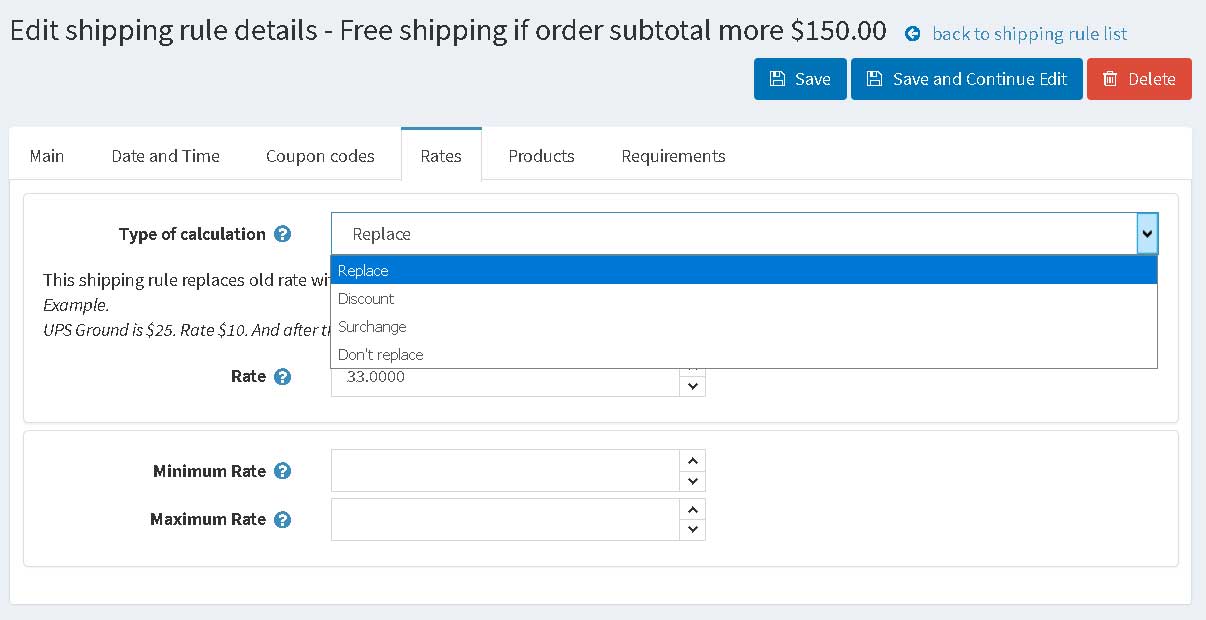**Detailed Caption:**

This image displays the "Edit Shipping Rule Details" section of an e-commerce control panel, where the website administrator can manage shipping rules. At the top of the page, the title "Edit Shipping Rule Details" is prominently featured. Beneath the title, a policy is stated: "Free shipping if order subtotal is more than $150." To the right, a navigation link labeled "Back to Shipping Rules List" is available.

In the upper right corner of the panel, there are three buttons for managing the shipping rule: a blue "Save" button, a blue "Save and Continue Edit" button, and a red "Delete" button.

Immediately below this section is the main area for editing the shipping rules. This control panel is used by the website owner to set parameters for shipping costs based on order details. 

The interface includes several tabs at the top: "Main," "Date and Time," "Coupon Codes," "Rates" (which is the currently selected tab), "Products," and "Requirements." The body of the page under the "Rates" tab includes several input fields and options.

The first option listed is “Type of Calculation,” which is a drop-down menu currently displayed with options: "Replace," "Discount," "Surcharge," and "Don't Replace." This section indicates that the administrator is setting or editing the shipping costs or rules for product orders on the website.